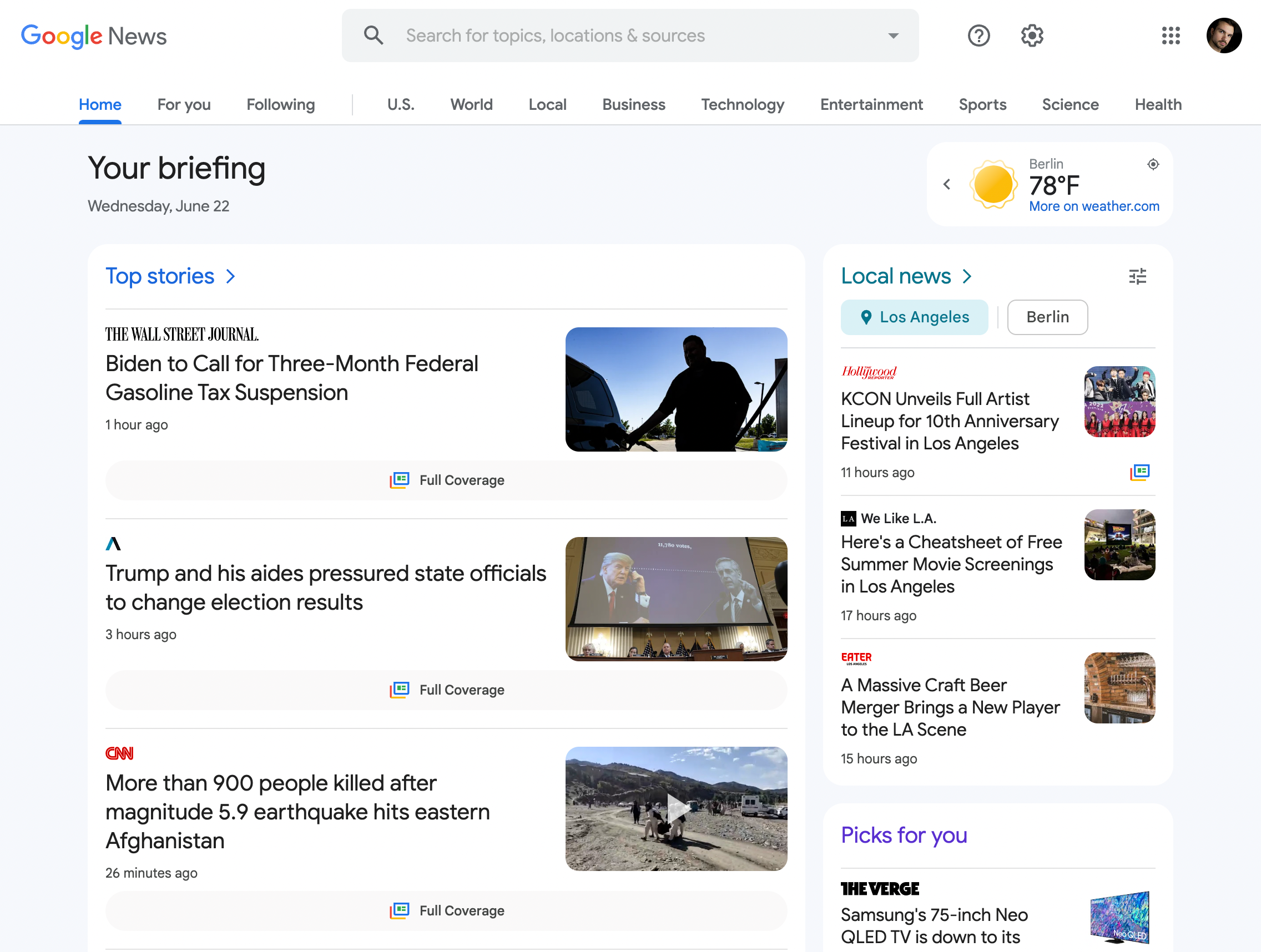A screenshot of the Google News homepage features a large search bar in the upper left corner and a circle profile image of a man's face against a black background in the upper right. Directly below the search bar, navigation options include "Home" in blue and underlined, followed by "For You," "Following," a vertical separator, and categories such as "US," "World," "Local," "Business," "Technology," "Entertainment," "Sports," "Science," and "Health." Just below "Sports," there's a white box displaying weather conditions with a yellow sun icon indicating a sunny day in Berlin with a temperature of 78 degrees Fahrenheit. Beneath this weather update, "Local news in Los Angeles" is highlighted in a blue rectangle next to "Berlin." On the left, "Top Stories" is labeled in blue, and above it, the date "Wednesday, June 22nd" appears with the heading "Your Briefing" at the top. The main news image depicts a man's silhouette pumping gas, accompanied by a headline from the Wall Street Journal: "Biden to call for three-month federal gasoline tax suspension." Another story headline mentions, "Trump and his aides pressured state officials to change election results," with a large screen image of Trump appearing to the left.